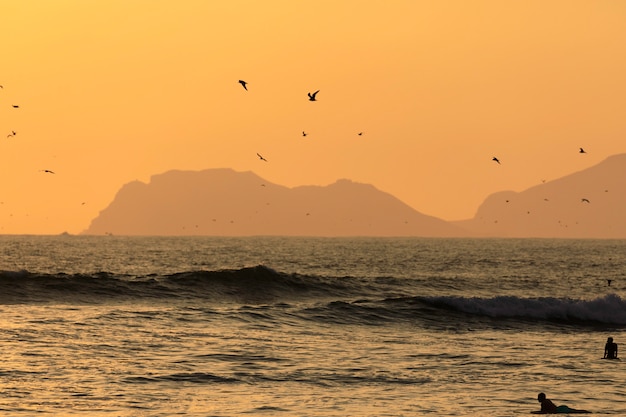The photograph captures a serene sunset over the ocean, with the sky painted in rich hues of orange and yellowish gold. The distant mountain range is veiled by a light haze, making its silhouette appear soft and out of focus. The water shimmers with the golden and orange reflections of the setting sun, creating a tranquil scene. In the bottom right corner of the image, the silhouettes of two figures are noticeable: one person lies prone on a surfboard or in shallow water, while another stands in waist-high water. Various birds, appearing as black silhouettes of different sizes, dot the sky, adding to the peaceful ambiance. Waves are calm with slight ripples, and a delicate shadow of a wave can be seen in the middle ground. The overall composition exudes a calm, almost ethereal quality as day transitions into night.